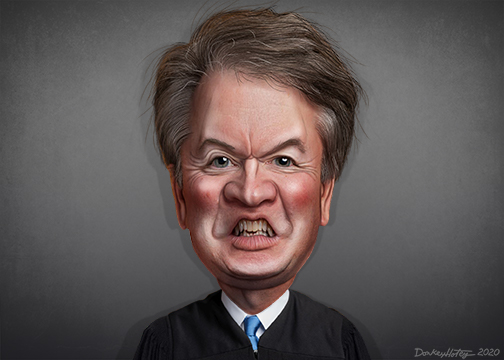In this image, we see a highly detailed and exaggerated caricature, likely of a political or judicial figure. The background is completely gray, accentuating the stark features of the subject. The figure is depicted as an old white man with a notably oversized head. His face is covered in deep wrinkles around his eyes, eyebrows, and chin, giving him a weathered appearance. Bright red cheeks stand out prominently against his pale skin.

The expression on his face is exaggerated with a wide nose, dimples around his nose, and an almost sneering, angry look. His teeth are depicted as tall, long, and slightly yellow, giving them a somewhat fang-like appearance. His hair is parted and brown, combed in a typical style for a political figure, which adds to the realistic yet caricatured feel of the drawing.

The attire consists of a black suit or judicial robe, a white dress shirt with a collar, and a light blue necktie. Only the upper torso of the figure is shown, focusing the viewer's attention on his exaggerated facial features. In the bottom right corner of the image, there is an artist's watermark that appears to start with a 'D' and a date marked as 2020, indicating the artwork's creation year.

Considering the exaggerated features and the context clues, the image likely makes a political statement, possibly depicting a Supreme Court justice such as Brett Kavanaugh or Neil Gorsuch, given the judge’s robe and the intense, almost sneering expression.